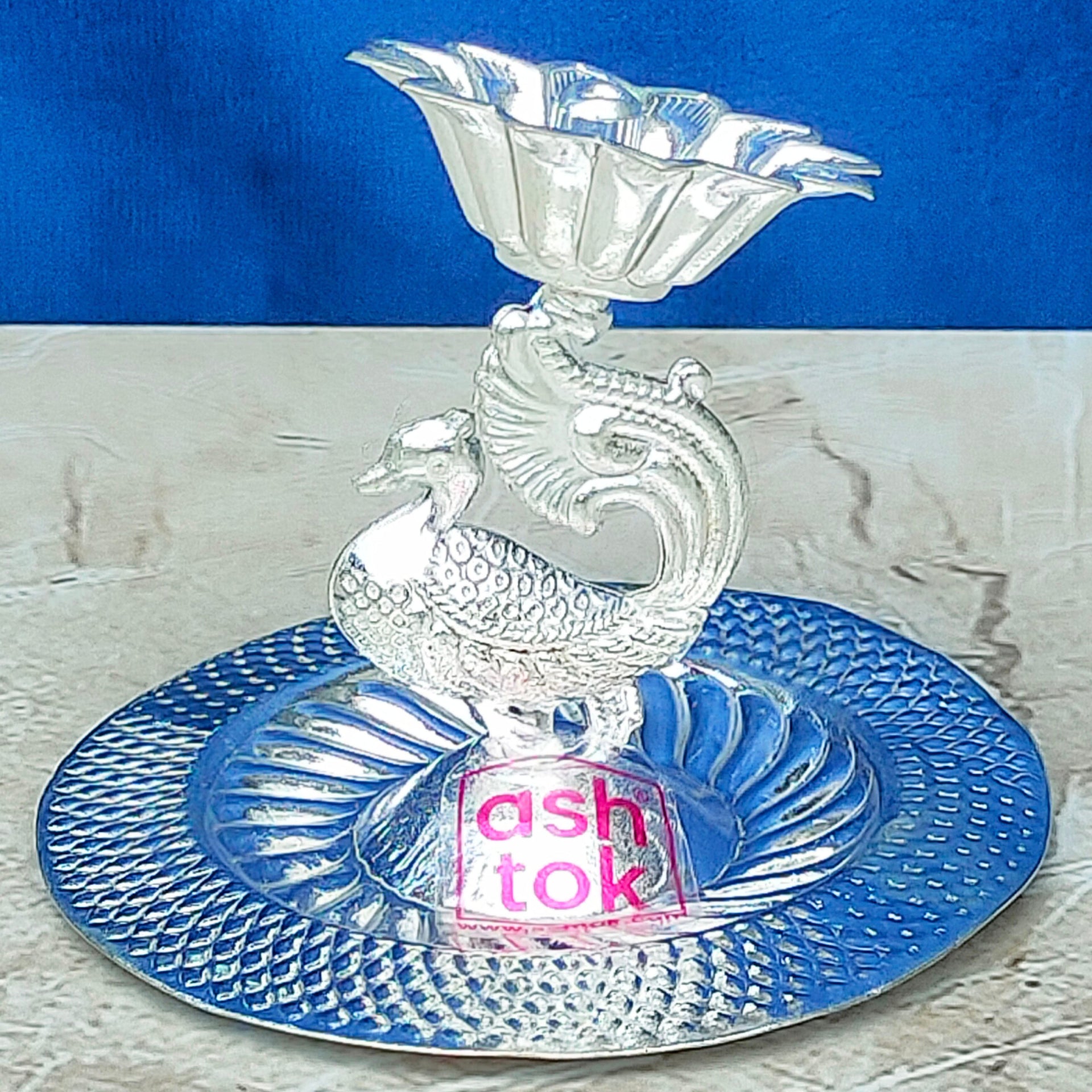The artwork is a detailed image featuring a sophisticated goblet ensemble. Starting with the background, the upper third is a textured deep mid-blue, while the lower two-thirds is a grayish white, complemented by a textured overlay that mimics the appearance of cracks or scratches. Dominating the bottom third of the image is a large blue plate adorned with silver scaling along the outer rim, contrasting with the flatter texture in the center. Perched in the center of the plate is an intricate sculpture of a peacock. The base of the goblet, reminiscent of bundt cake texture, gracefully transitions into the peacock, whose head faces left with ornate detailing. The peacock's tail rises upwards, morphing into a flower-shaped bowl, presumably the goblet's drinking vessel. The entire goblet appears to be made of clear, glass-like material with silver embellishments. Additionally, there is a mention of inscriptions in pink letters saying "ash top" or "Ash, A-S-H, talk" near the outer edge of the plate. The scene is set against a white table, with the blue background contributing to the overall vibrant and elegant presentation. This elaborate setup projects a sense of luxury and would make a delightful gift for enthusiasts of fine art.